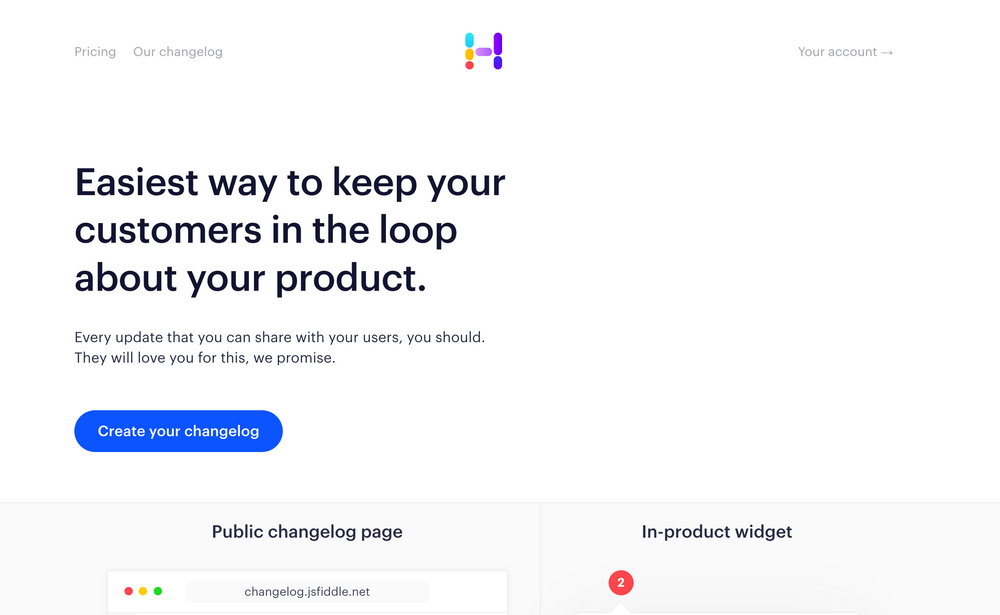This image is a screenshot of a website or web application, characterized by a clean and minimalistic design with a predominantly white background. 

At the top-left corner, there are two menu items labeled "Pricing" and "Changelog," written in small, light gray, sans-serif text in sentence case. A large empty space separates these from the center-aligned logo.

The logo itself is an abstract design in the shape of the letter "H," comprised of various colorful oval lines. The colors included are cyan, golden yellow, orange, red, purple, and violet.

On the top-right corner, there is an account icon represented by a small arrow pointing to the right. Directly below this area, there is some white space.

The main content begins with a prominent headline on the left side, written in the largest font size (approximately size 41). The text reads, "Easiest way to keep your customers in the loop about your product." Below this headline, there is a paragraph of smaller text stating, "Every update that you can share with your users, you should. They will love you for this, we promise."

Further down, there is a blue button with rounded edges that says, "Create your changelog." Beneath this button, the image cuts off, but there appears to be a preview or description of the product's features. The preview is divided into two sections against a light gray background. The left section is titled "Public Changelog Page," displaying the top part of a browser with the URL changelog.jsfiddle.net. The right section is titled "In-Product Widgets," featuring a red circle with the number two inside it, presumably indicating notifications or updates.

Overall, the design is clean and user-friendly, guiding the viewer's eye through a well-structured layout.